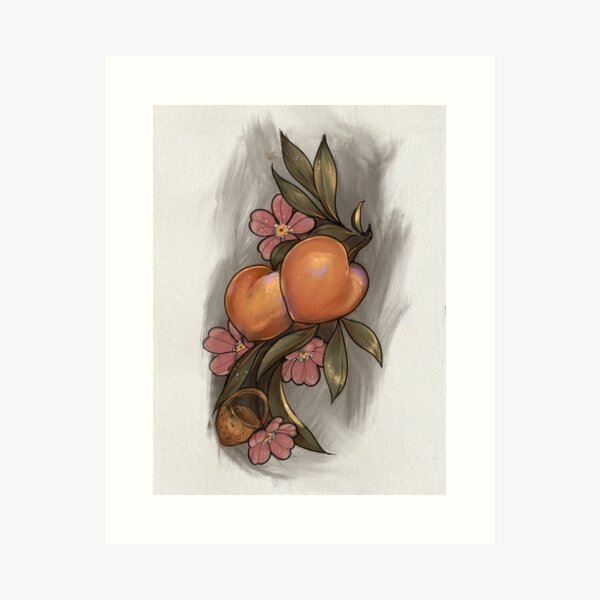The illustration, set against a cream-colored background that varies from grey to a peachy light grey, depicts a lush plant with an abundance of green leaves extending to the top and bottom of the image. Nestled at the heart of the plant, two fruits that resemble peaches or nectarines are shaped like hearts. Scattered amidst the foliage are four delicate flowers with pink petals and white and yellow buds. At the bottom left, there is a small brown nut and what appears to be a tiny basket. The plant itself casts subtle, dark shadows, adding depth to the computer-generated or cartoon-like drawing. The outer frame of the illustration consists of a light grey square, transitioning into a light green rectangle, and finally a darker green rectangle encompassing the vibrant scene of fruits and flowers.